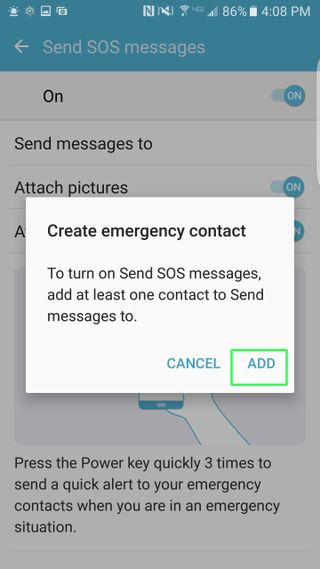The image is a screenshot of a settings interface on a smartphone, likely meant for configuring emergency message features.

In the top left corner, there's an icon that resembles a bulb, possibly indicating a source of light or idea. Adjacent to it, there's a picture icon and a square icon labeled "NFC". 

Further down, there are labels for "Speakers" and "Wi-Fi," although the former is not clearly visible and appears to be toggled off, while the battery charge is shown at 86% with the current time displayed as 4:08 PM.

A left arrow icon is present, likely indicating a back navigation option. Below it, "Send SOS messages" is highlighted within a blue bar. A blue circle suggests that the toggle for sending SOS messages should be turned on. 

To activate this feature, at least one emergency contact must be added. The interface offers an option to "Create Contact" to fulfill this requirement. A red border with white and blue text indicates additional instructions or alerts.

The screen further details the function: "Press the power key quickly three times to send a quick alert to emergency contacts when you are in an emergency situation." This instruction is bordered in blue to emphasize its importance.

Behind this active window, there seems to be a greyed-out screen, indicating that the current settings window is prioritized.